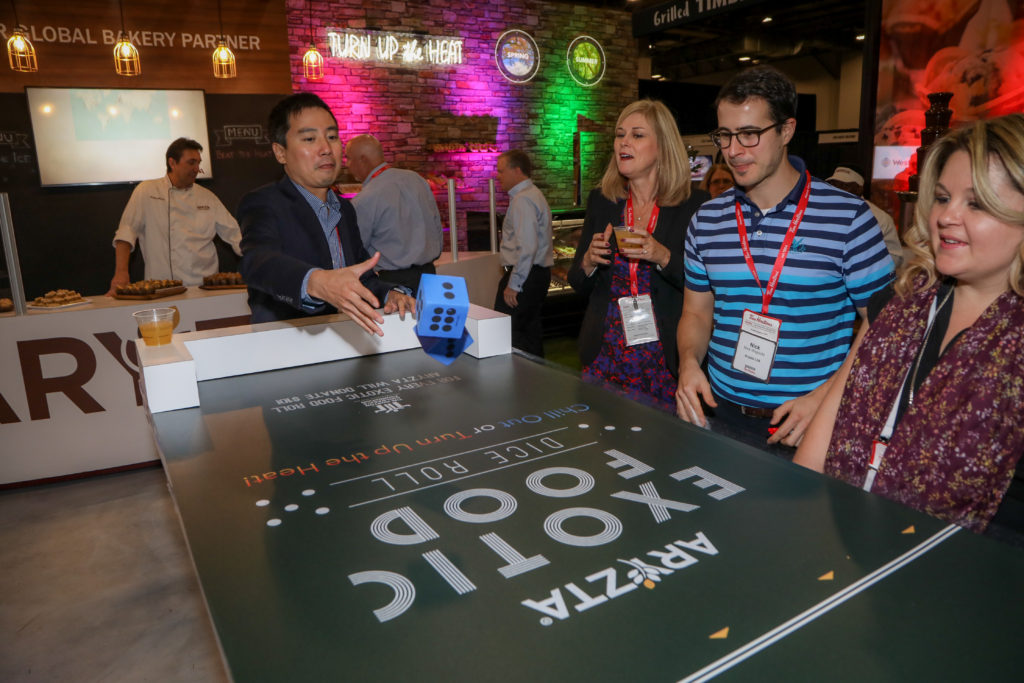In this vibrant indoor photograph, reminiscent of a lively eatery or bar, we see a bustling gathering or party unfolding. The centerpiece is a long flat table in the foreground, adorned with text that reads "ARYZTA Exotic Foods Dice Roll. Chill out or turn up the heat." This text is initially upside down in the image. At the end of this table, a man of Asian descent is captured in the dynamic act of rolling a large blue die, with a drink placed beside him. Adjacent to him on the right, three onlookers—a man flanked by two women—stand attentively, each adorned with lanyards, suggesting they are attendees of this event.

The backdrop is equally engaging, featuring a brick wall bathed in atmospheric lighting of green, purple, and pink hues. Positioned to the left in the background, a male chef, donned in a pristine white jacket, stands in front of a screen with the illuminated sign "Global Bakery Partner" above it. In front of the chef's counter, laden with trays of enticing baked goods, two men are actively engaging with him, presumably discussing or sampling the offerings. Farther to the right, another neon sign brightly proclaims, "Turn up the heat," contributing to the lively and festive ambiance of the scene.